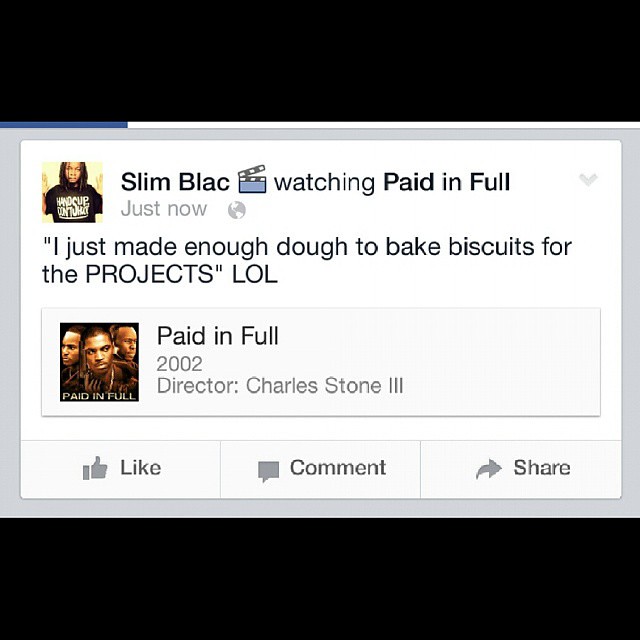A detailed descriptive caption based on the combined and cleaned-up information is as follows:

A screenshot of a Facebook post by Slim Black, showing a social media post with two images. The user profile shows a young black man with dreadlocks, wearing a black t-shirt with white writing. The post's text reads, "Slim Black watching Paid in Full just now. I just made enough dough to bake biscuits for the projects, LOL," indicating he recently watched the film and humorously commented on it. The post includes a thumbnail image of the 2002 movie "Paid in Full," directed by Charles Stone III, with three African American male headshots on the cover. The post is interactive with icons for liking, commenting, and sharing, and is framed by large black bars at the top and bottom, creating a perfectly square image space.